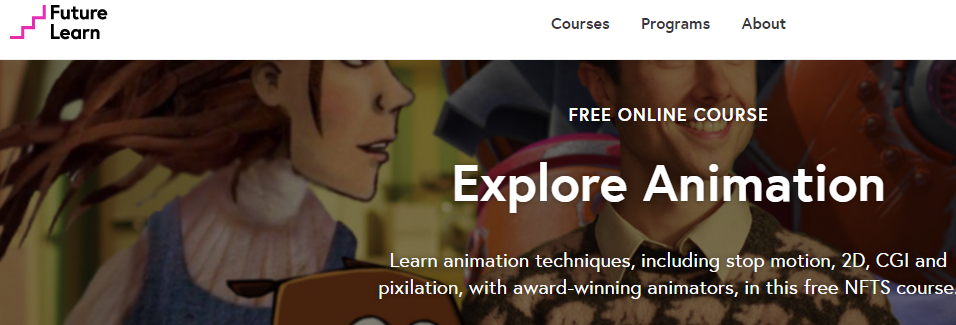This is an advertisement for Explore Animation by FutureLearn. The ad features a pair of pink stairs on a white background. The word "FutureLearn" is prominently displayed in black letters above the stairs. Surrounding the text are links for "Courses," "Programs," and "About." Below this, in a rectangular box, there are charming, hand-drawn figures of a girl with flyaway hair and a boy. The caption reads, "Free Online Course: Explore Animation. Learn animation techniques, including stop motion, 2D, CGI, and pixelation with award-winning animators in this free NFTS course." The background is filled with various children-themed illustrations, suggesting that the course may be suitable for young audiences. The animators have skillfully rendered the children and their playful surroundings, effectively capturing the spirit of the topic.